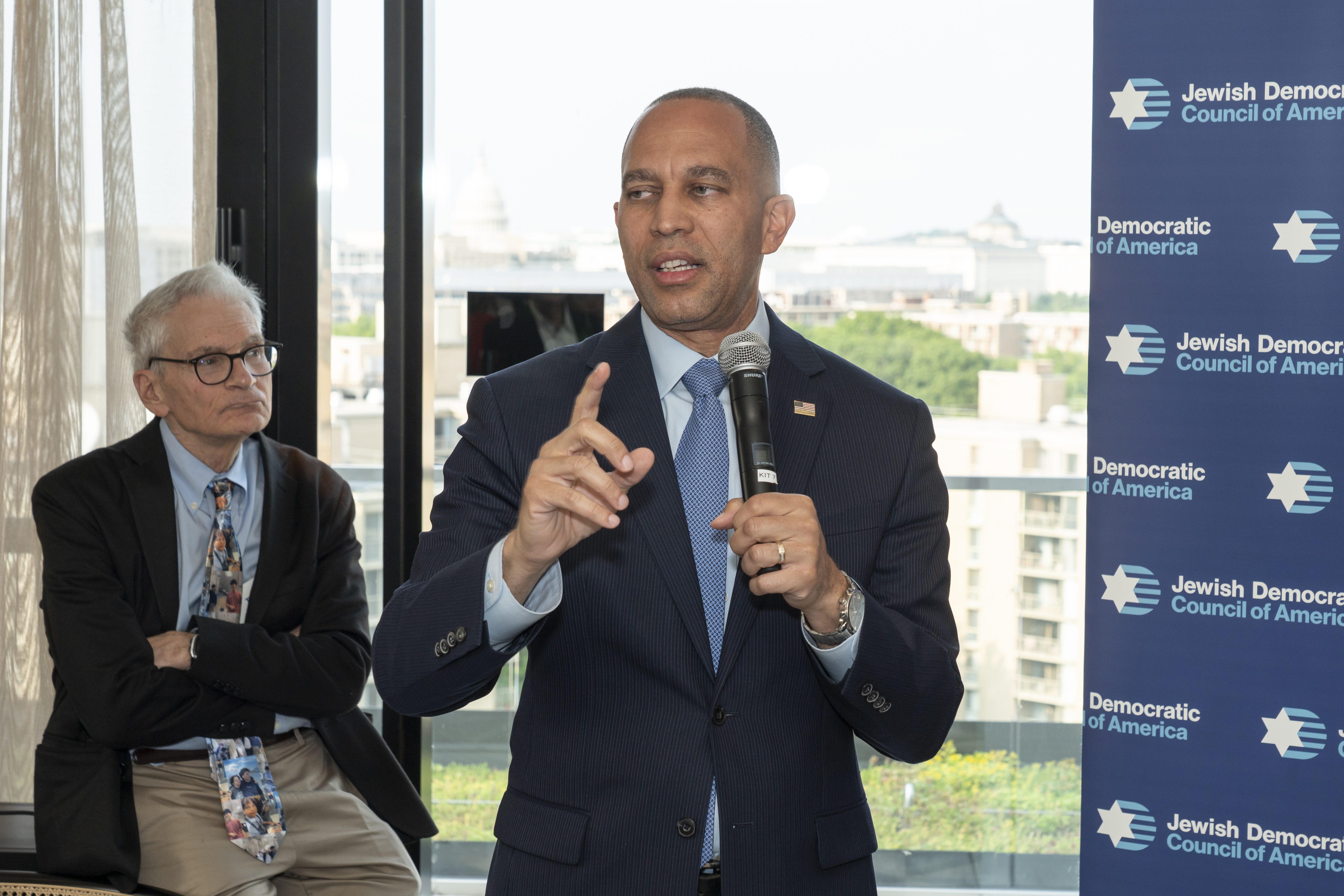The photograph captures a man speaking at an event for the Jewish Democratic Council of America, as indicated by the banner on the right side of the image. The man, who appears to be in his mid-40s, has medium-toned skin, very short hair, and no facial hair. He is wearing a well-fitted, navy blue business coat with an American flag lapel pin, a light blue button-up shirt, and a solid medium-blue tie. He is articulated with his left hand holding a black microphone and his right index finger pointed upwards in a gesture. His body faces forward, but he looks towards the left.

In the background, daylight filters through a large window, revealing a cityscape of tall buildings. To the left, an older gentleman, probably in his 70s, sits on a table. He has short grayish-white hair and wears plastic black-rimmed glasses. His outfit includes medium-colored khaki pants with a brown leather belt, an open black suit jacket, a light blue button-up shirt, and a tie adorned with various photographs of people. This man sits with his arms crossed and gazes intently, possibly at someone unseen in the photograph.

The juxtaposition of the engaged speaker and the pensive older man, along with the urban backdrop, creates a dynamic scene that hints at a formal gathering or conference.